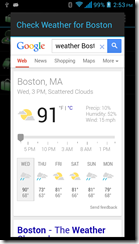In this image, we see a somewhat blurry screenshot set against a black background, featuring a weather update for Boston, Massachusetts. At the top, all bars of the Wi-Fi icon indicate a strong connection. 

The main text, displayed in blue, reads "Check weather for Boston." Below this, there is a white rectangular box containing detailed weather information. The text inside the box reads:

"Google weather, Boston, Massachusetts, Wednesday, 3 p.m., scattered showers." An icon depicting a sun partially obscured by two clouds symbolizes the weather conditions. The temperature is shown as 91°F, with a 10% chance of precipitation, 52% humidity, and wind speeds of 15 miles per hour.

A gray horizontal line separates different sections of the forecast. Following this line, the same weather details for 3 p.m. on Wednesday are repeated: "Boston, Massachusetts, Wednesday, 3 p.m., scattered showers," along with the same icon and weather statistics.

Another gray horizontal line lies below this repetition, separating the hourly forecast from the weekly outlook. The days of the week are listed in succession: Wednesday, Thursday, Friday, Saturday, Sunday, Monday, Wednesday, and Tuesday. Next to these days are brief weather summaries with high temperatures: Wednesday (90°F), Tuesday (high of 73°F), Friday (85°F), and Saturday (81°F).

Overall, the screenshot provides a comprehensive weather update for both the immediate and forthcoming days.